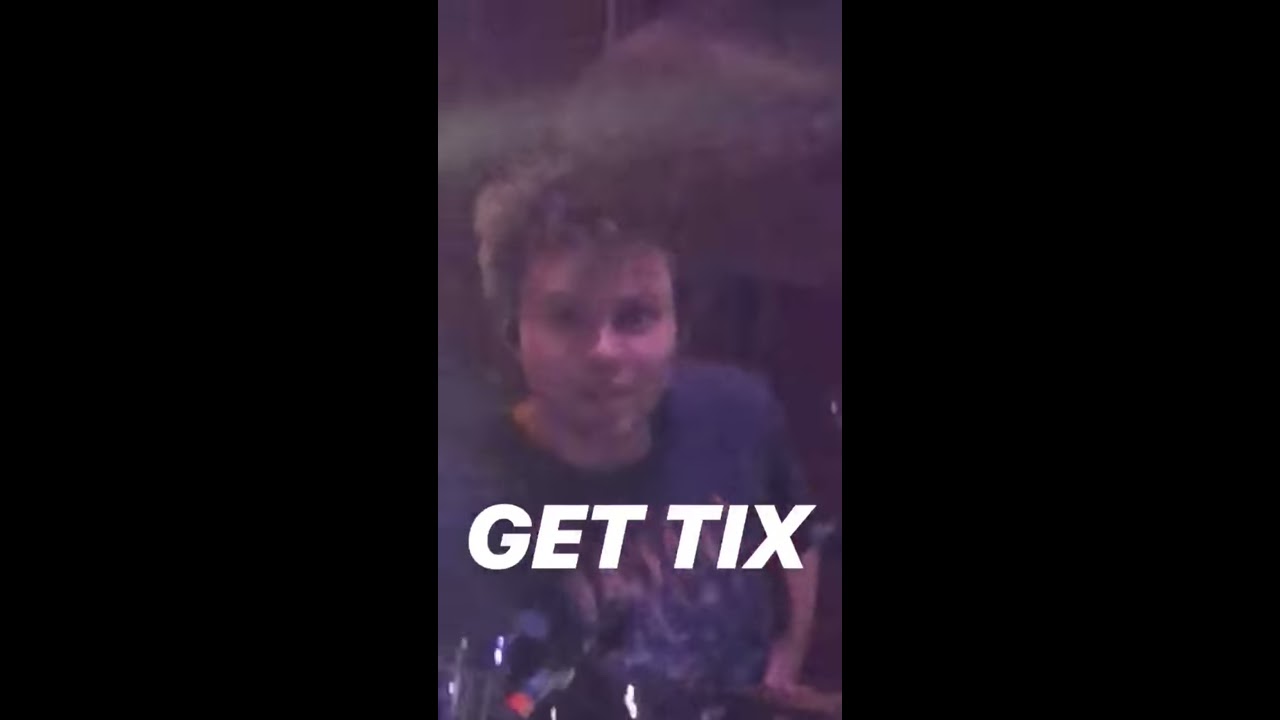A color portrait image in a vertical cell phone orientation features a man with curly, unruly brown hair wearing a dark t-shirt, potentially navy or black, with some brown and white decoration on the front. He is positioned in the center of the photograph, surrounded by black bars framing either side. The lighting from the left side creates highlights in his hair, while the overall image appears hazy and blurry, obscuring fine details. The man's mouth is slightly open and his eyes wide as he looks into the camera, giving an impression of a partial smile. The lower third of the image contains bold, white, all-capital block text reading "GETTIX," which partially covers his chest. The background behind him is indistinct and brownish, with maybe a drinking glass faintly visible on the left.